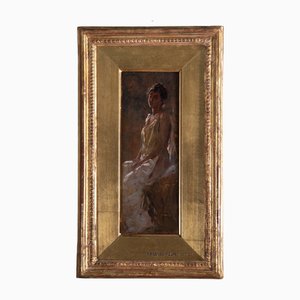The image depicts a small, framed painting, roughly two inches high by two inches wide, set against a light gray or bluish-gray wall. The painting itself is a narrow, vertically oriented rectangle, measuring approximately three-quarters of an inch high by a quarter of an inch wide, encased in an ornate gold frame with beveled edges and intricate detailing that includes raised circles around the inner part. Central to the painting is a woman with dark hair, styled in a large bun, sitting and facing left. Her head is slightly tilted toward the viewer, and she has a brown skin tone. She wears a long, sleeveless robe, gold around the torso, and transitioning to white at the bottom. Her hands rest in her lap, though finer details are difficult to discern due to the image’s small size. The composition is such that her feet are near the bottom of the painting, with a small gap above her head to the top edge, and the right side of the painting cuts off behind her back, while the left side is near her knees, suggesting a close-cropped view.